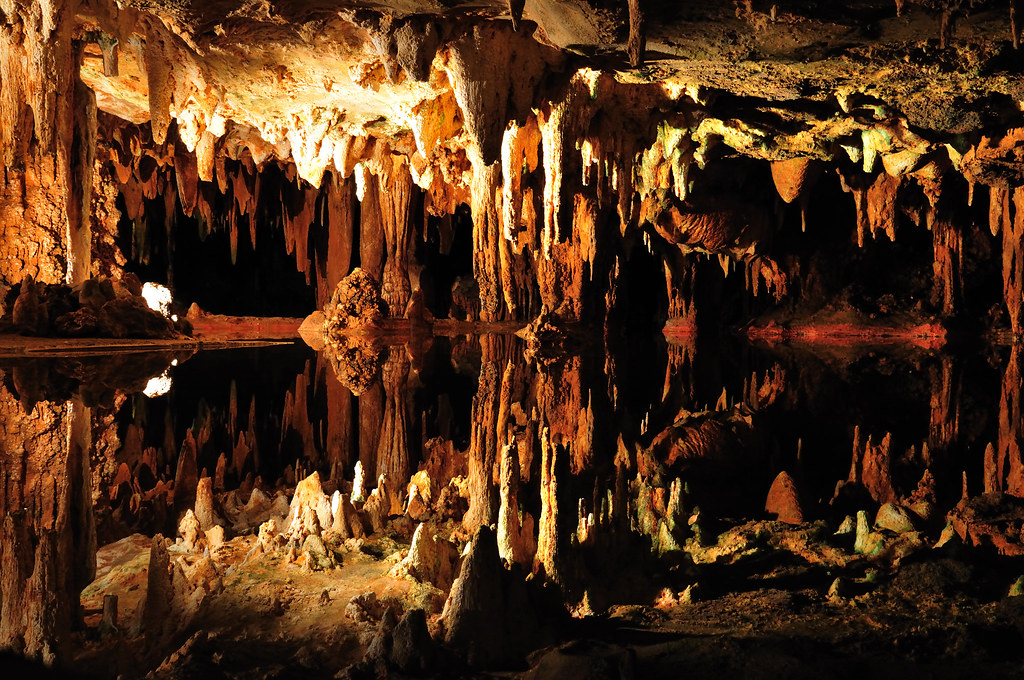The image depicts a mesmerizing cave with an ethereal and almost surreal quality. The cave's ceiling, adorned with numerous jagged stalactites and overhanging rocks, is perfectly reflected in the still water below, creating a flawless mirror image that doubles the scene’s intensity. The water is so calm and clear that it becomes nearly invisible, enhancing the illusion of symmetry within the cave. The cave's interior is cloaked in darkness, with the stone surfaces exhibiting earthy yellow hues that contrast sharply with the black surroundings. The uncanny precision of the reflection makes it hard to distinguish the boundary between the actual cave and its mirrored counterpart, lending the scene an almost dreamlike, trippy appearance. Whether a natural wonder or a digitally created image, this breathtaking visual presents a fascinating and thought-provoking spectacle.